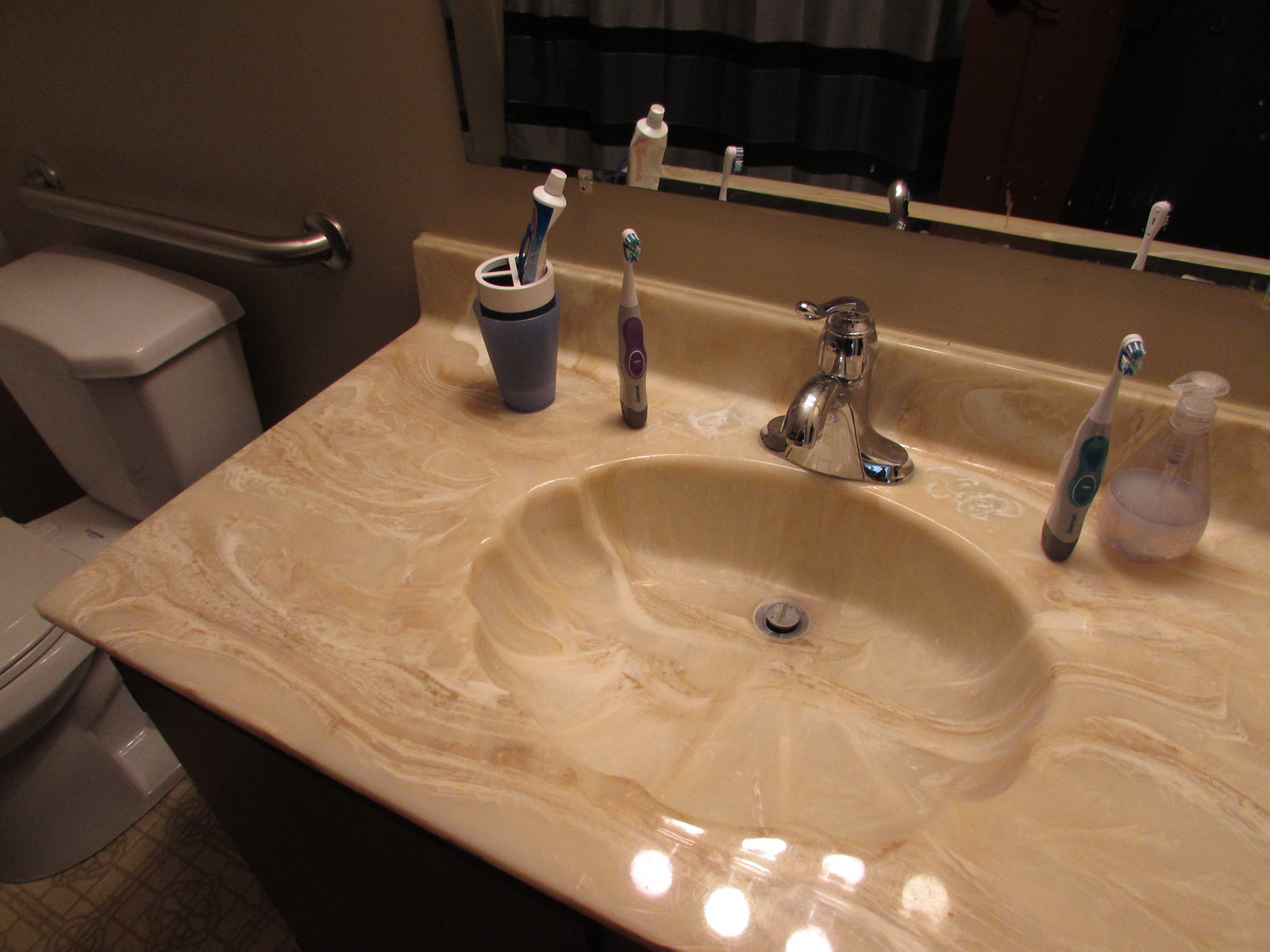This photograph captures a vintage bathroom sink, likely from the 1980s or 1990s, featuring a distinct scalloped shape that gives it an oval yet slightly oblong appearance. Both the sink and the countertop are crafted from the same material, exuding a glossy, plastic-like finish with a marbled pattern that resembles spilled coffee creamer. The faucet is a practical and streamlined silver fixture with a single lever handle.

Adjacent to the sink, there is an assortment of personal items. On either side of the sink, electric toothbrushes stand ready for use. On the right, a partially filled soap dispenser containing a light, semi-transparent liquid is placed conveniently for handwashing. To the left, a purple cup with a white holder at its top is visible, along with a tube of toothpaste emerging from it.

A mirror is mounted a few inches behind the sink, reflecting the upper part of the room. Above the mirror, four round bulbs contribute ample lighting, their reflections also visible on the countertop below, which enhances the brightness of the space.

To the left of the sink stands a white toilet, complemented by a grab bar installed above it, providing safety and support. The walls are painted a medium beige, creating a warm and neutral backdrop for the fixtures. Overall, this image evokes a nostalgic sense of home, reminiscent of a bygone era.